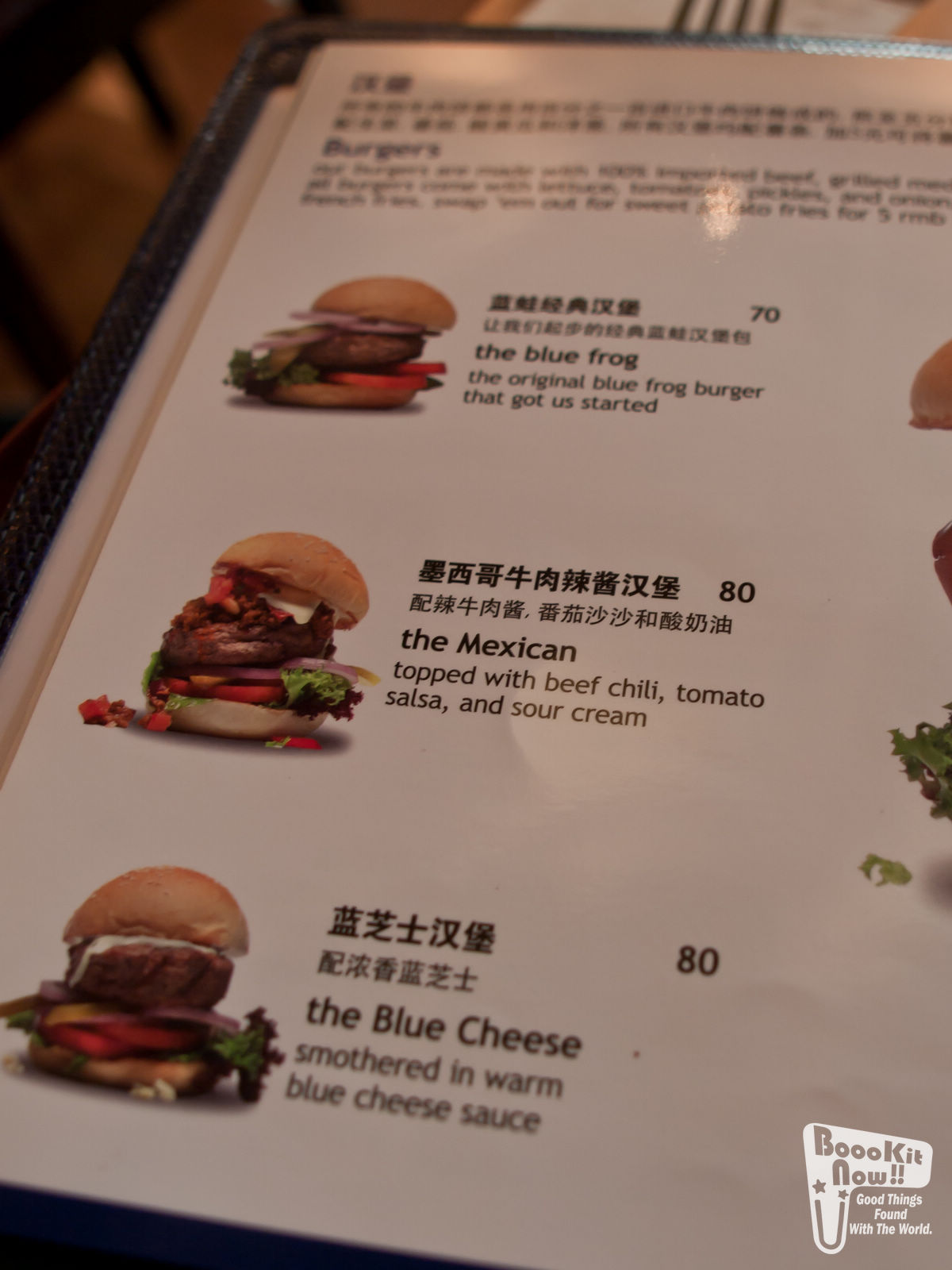The image showcases a menu predominantly featuring Chinese characters with accompanying English translations. In the bottom right corner, the text "Book it now" is displayed, possibly indicating a reservation option. This text is styled with a U-shaped design, with stars positioned above the ends of the U. The U-shaped design is rendered in a putty color against a white background. Additionally, the phrase "Good things found with the world" is prominently featured on the menu.

The menu highlights several items, including:

1. The "Blue Frog," touted as the original Blue Frog burger, a signature item that initiated the menu.
2. A burger called "The Mexican," which includes toppings such as beef chili, tomatoes, salsa, and sour cream.
3. The "Blue Cheese" burger, described as being smothered in a warm blue cheese sauce.